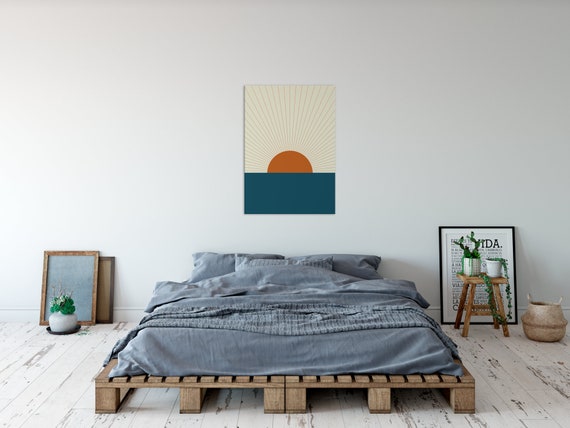The image depicts a minimalist bedroom with a low bed constructed from four wooden pallets, creating a rustic yet intentional look. The bed features a thin mattress hidden beneath a partially made, dusty blue-gray comforter and sheets, accompanied by matching pillows. It rests on a worn, white-painted wooden floor. The stark white wall behind the bed serves as the backdrop for a striking, vertically rectangular painting of a stylized rising sun over water. This artwork features a navy blue lower half, a cream upper half, and a dark rust orange sun with perfectly radiating rays. Flanking the bed on either side are several picture frames leaning against the wall, and a stool repurposed as a nightstand holds a plant and a mug, with another planter beside it. On the other side, a white pot containing a green plant further enhances the serene, naturalistic ambiance.